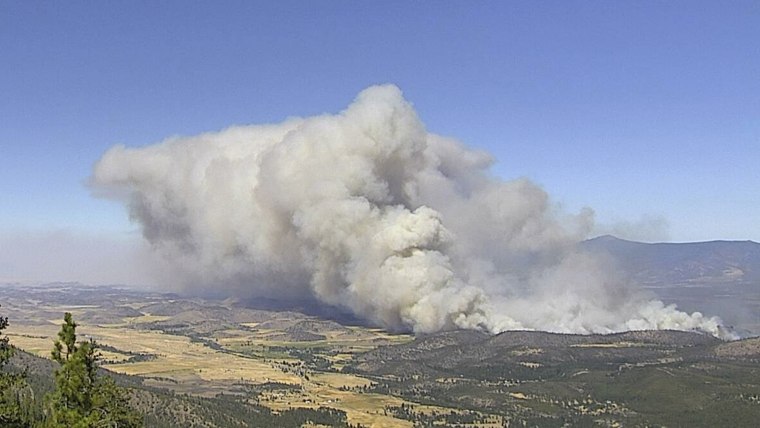The image is a high-angle, outdoor photograph taken from an elevated position, possibly a mountain, overlooking a vast landscape. In the foreground, a couple of pine trees are visible on the left, with expanses of green fields and patches of brown dirt and hills below. Dominating the scene, massive plumes of thick, gray smoke rise from a large wildfire in the valley, obscured by the hills. The smoke, varying in shades of white to medium gray, billows intensely, suggesting the fire is extensive and recently ignited. Despite the large amount of smoke, no flames are visible. Beyond the smoke, the landscape features a mountain range and agricultural land, all under a bright blue, cloudless sky.